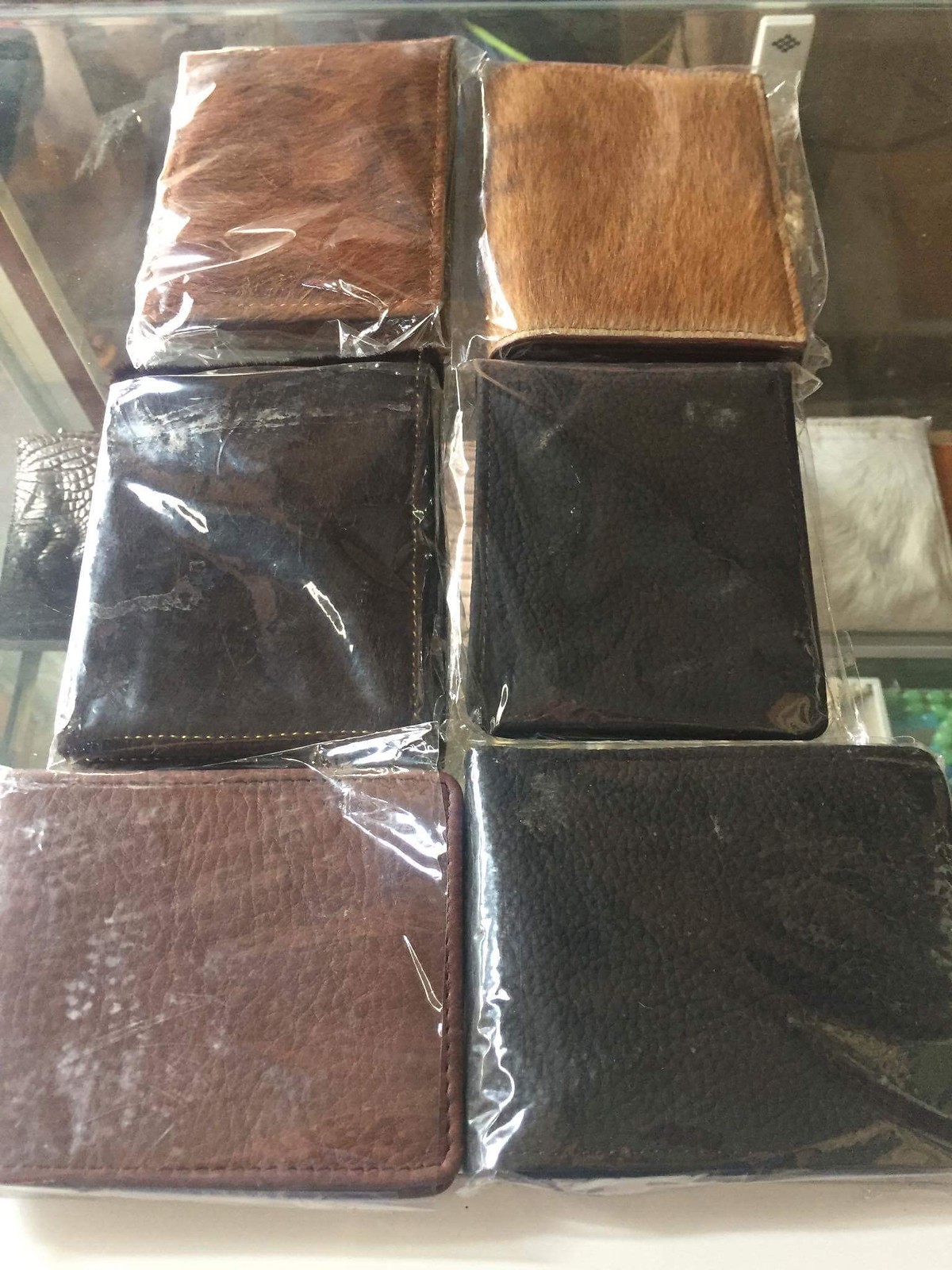This indoor photograph showcases six leather wallets displayed on a see-through glass countertop. Each wallet is encased in clear plastic wrap. On the top row, positioned vertically, there is a dark brown wallet still in its plastic packaging on the far left, and next to it, a lighter brown wallet, resembling a rawhide shade. On the second row, the left wallet is black with distinct white stitching around its edges, while the one adjacent to it is a square-shaped black wallet, both in plastic. The bottom row features a dark brown square wallet on the left and another black square wallet on the right, both still in plastic wraps. The wallets appear to be a mix of bi-fold and tri-fold designs, and are possibly made of vinyl leather. Underneath the glass countertop, various indistinguishable items, potentially other wallets, are visible but obscured by the displayed wallets on top.